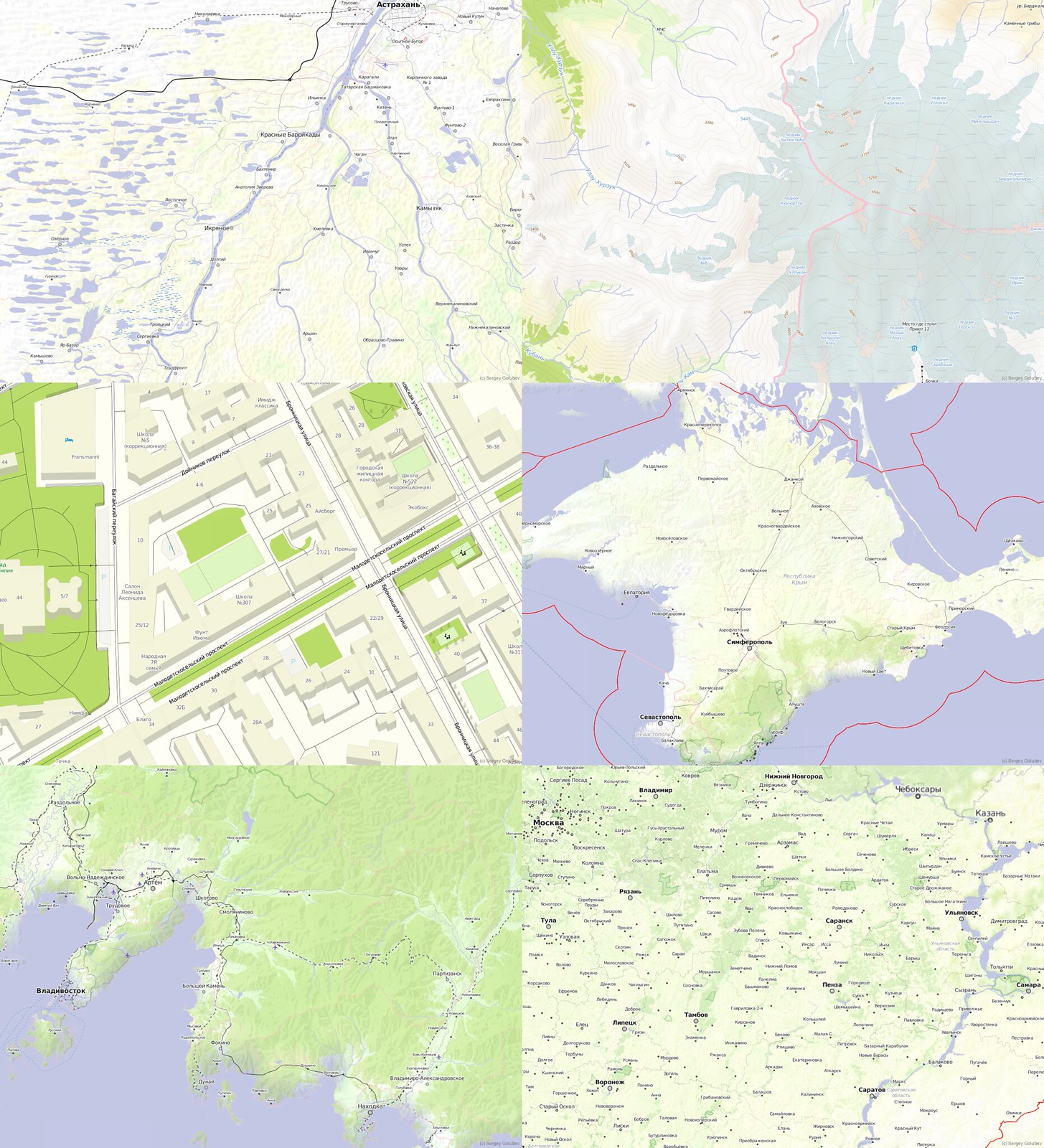This image features a mosaic collage of six distinct maps, each varying in zoom level and region depicted. All maps share a palette of pale colors including white, yellow, blue, and green, and are characterized by intricate yet hard-to-read details due to the small, often foreign text in black. 

In the top left corner, the map captures a landscape populated with numerous small lakes. Adjacent to it in the top right, the map shows an icy or mountainous region devoid of city markings. The middle left map displays a detailed street grid, likely portraying an urban area, while the map next to it presents an island surrounded by blue ocean waters, dotted with place names. 

The bottom left map reveals a rugged coastline with a trail or road navigating through diverse terrains highlighted in green and blue tones. Finally, in the bottom right, the map depicts a complex topographical view with a river coursing along the right side, showing varied gradients in green hues and dense city names scattered throughout the landscape. The overall composition illustrates diverse geographic features, ranging from urban grids and road networks to natural landscapes and topographical variations, providing a multidimensional representation of different locales.